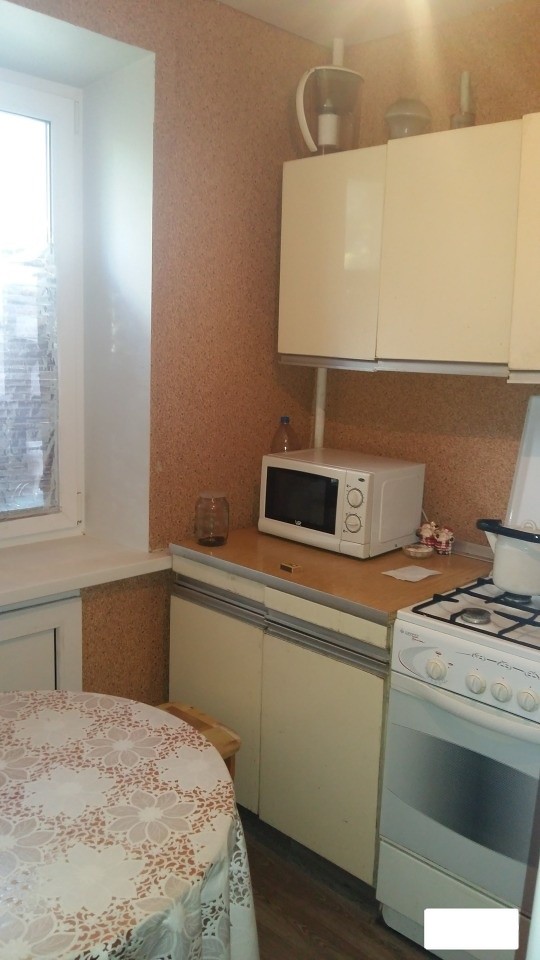This color photograph captures the corner of a cozy kitchen bathed in natural light. The walls are painted a warm tan or peach color, enhancing the inviting atmosphere. Dominating the right side, white cabinets with silver handles and a brown wooden countertop host a small, white countertop microwave with a dark window. Above the microwave are three additional cabinets used for storage, with various indistinguishable items resting on top. Adjacent to the microwave is a white gas stove featuring black wrought iron racks and four knobs.

To the left, a large window with open shades allows sunlight to pour into the room, highlighting a small, round dining table draped in an elegant white lace tablecloth patterned with delicate floral designs. The table shares the space with wooden stools, adding to the kitchen's charm. The countertops and cabinets create a cohesive, organized look ideal for a compact, functional kitchen area.